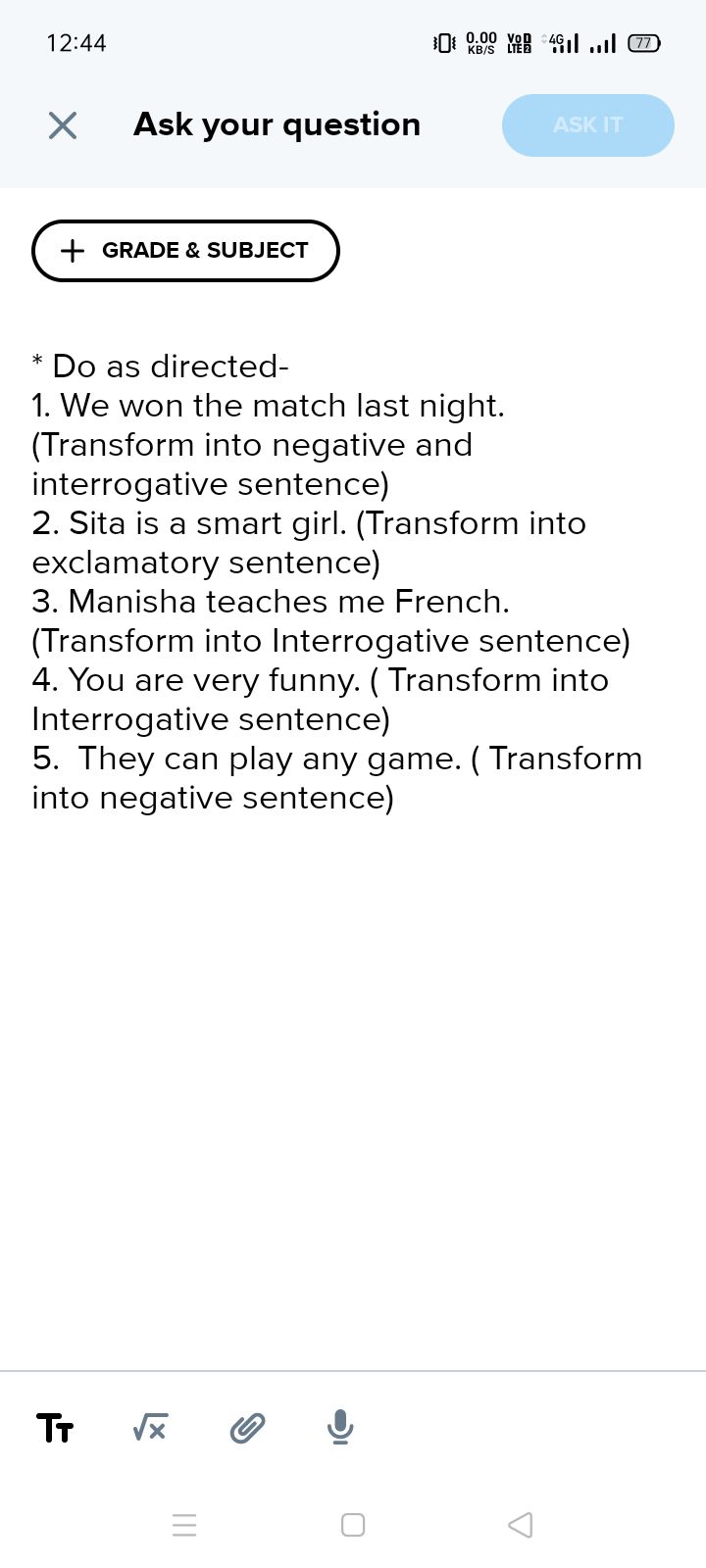This image is a screenshot of a smartphone display showing a user interface with detailed elements and controls. 

- The time on the clock is 12:44, with the phone set to vibration mode.
- The data transfer rate is 0.0 KB/s, indicating inactivity in internet data usage.
- The carrier status shows “LTD” with a 4G connection, providing full signal strength represented by four bars. 
- The battery level is at 77%.
- At the top-right corner, there's a close icon (X).

Below, prominently featuring:
- A bold prompt stating, "Ask your question."
- Next to it, a blue button labeled "Ask it".

Further down, there is a capsule-shaped outline with a plus symbol followed by text inputs labeled "Grade" and "Subject". An asterisk guides users to "Do as directed".

Numbered tasks are presented for transformation:
1. **We won the match last night.** *(Transform into negative and interrogative sentences)*
2. **Sita is a smart girl.** *(Transform into an exclamatory sentence)*
3. **Manisha teaches me French.** *(Transform into an interrogative sentence)*
4. **You are very funny.** *(Transform into an interrogative sentence)*
5. **They can play a game anytime.** *(Transform into a negative sentence)*

Significant white space follows these tasks, leading to a thin bar with toolbar options:
- A large uppercase "T" and a smaller uppercase "T"
- A square root sign with an "X" inside it
- A paperclip icon for attachments
- A microphone icon for voice input

The background of this section is white, and beneath it, in light gray, are the three standard buttons for the navigation bar against the same white background.